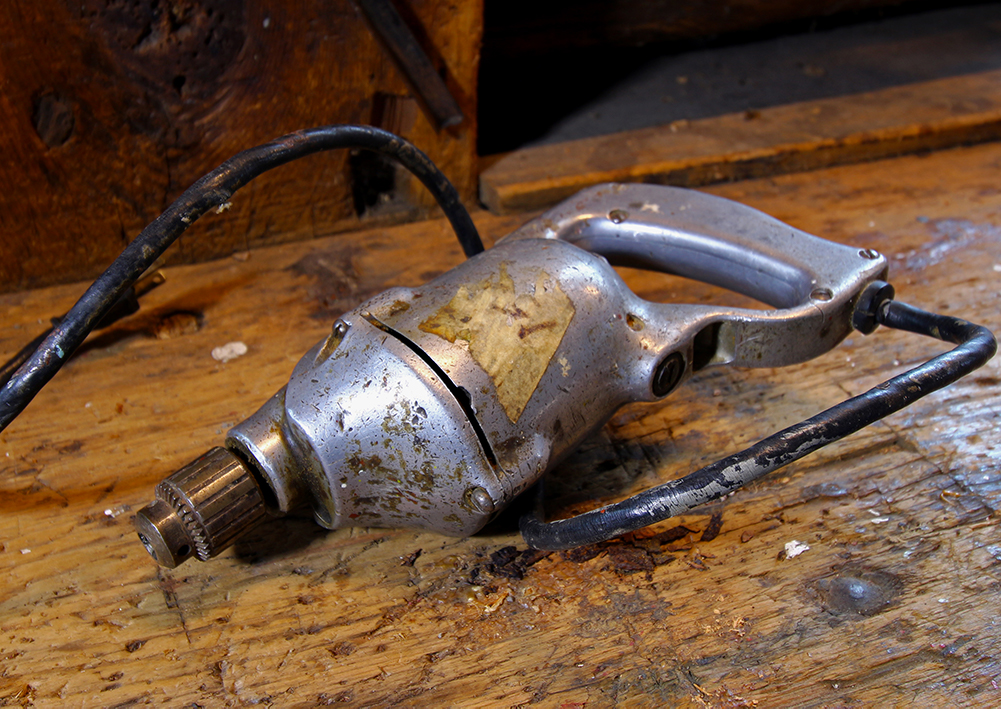The photograph showcases a heavily used, old electric drill resting on a weathered wooden workbench. The workbench, made of tan wood, is scarred with numerous scuff marks, gouges, and discolorations, indicative of extensive use. The drill, painted gray with a black metal drill bit area, bears the remnants of a faded sticker in the center of its body. Three screws are visible on the front, holding the engine casing together. An attached black cord extends from the base of the thick metal handle. Despite its wear and tear, including the sticker worn down to a gray tatter and the paint-splattered cord, the drill remains identifiable and functional, positioned with its front pointing towards the bottom left corner of the image. The backdrop reveals a wood wall in the upper left, adding to the rustic workshop setting.